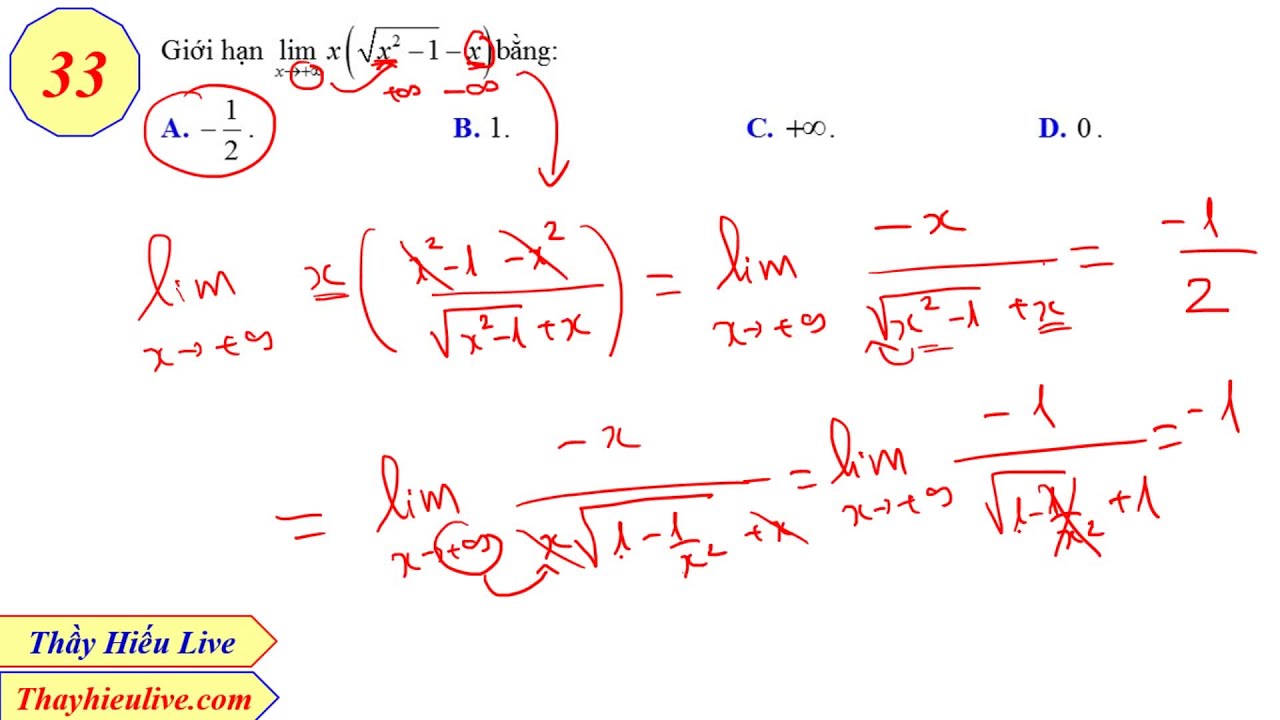The image depicts a complex mathematical equation written in red text on a white background, with a mixture of algebraic and possibly advanced mathematical symbols. In the upper left corner is a yellow hexagonal shape with blue edges, containing the red number "33" at its center. To the right of this shape, black text poses a mathematical problem. Below this, multiple potential answers (A, B, C, D) are listed, with A providing the value -1/2, B being 1, C given as positive infinity, and D as 0. The correct answer is indicated by the circling of option A. Additionally, two pentagon shapes are located in the bottom left corner, with blue text in the top pentagon and red text in the bottom one. At the bottom of the image, there is text in a foreign language, alongside the name “ThuHuLive” and a web address “ThuHuLive.com,” suggesting the source or presentation of the content.